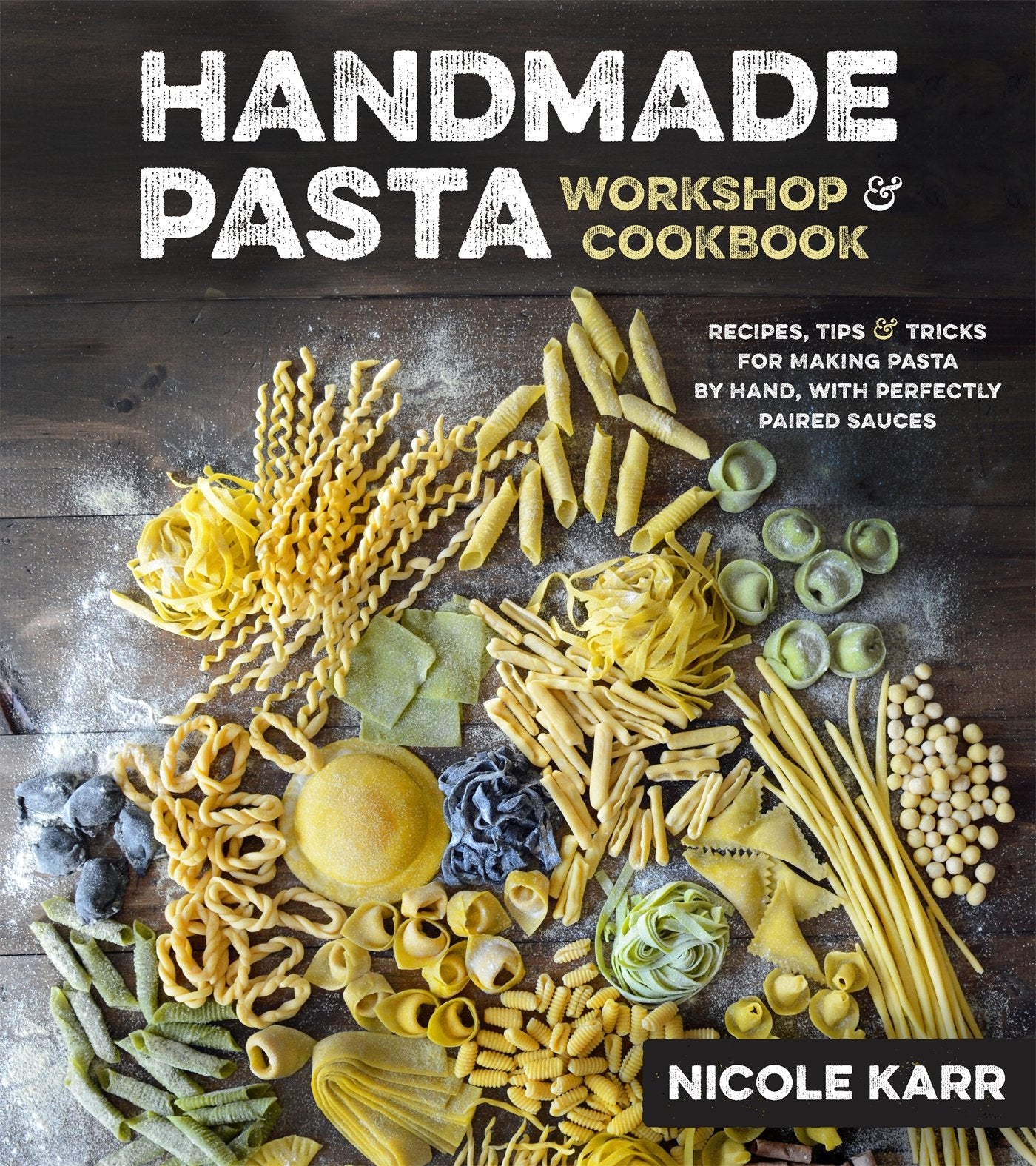The cover of the "Handmade Pasta Workshop and Cookbook" by Nicole Carr features a dark gray background with vibrant text. "Handmade Pasta" is prominently displayed at the top in white letters, accompanied by "Workshop and Cookbook" in yellow. Below, a descriptive blurb in white text offers insights into the contents: "Recipes, tips, and tricks for making pasta by hand with perfectly paired sauces." At the bottom right, Nicole Carr's name appears in white within a dark brown rectangular box.

The main image showcases an assortment of pasta varieties artfully arranged in a circular pattern on a wooden table with visible wood grain and slots. Various shapes and sizes of pasta, including penne, tortellini, gnocchi, ravioli, and spaghetti, are displayed in clusters. The pasta colors range from traditional yellow to light green and purple, while a dusting of flour adds an authentic touch to the scene.